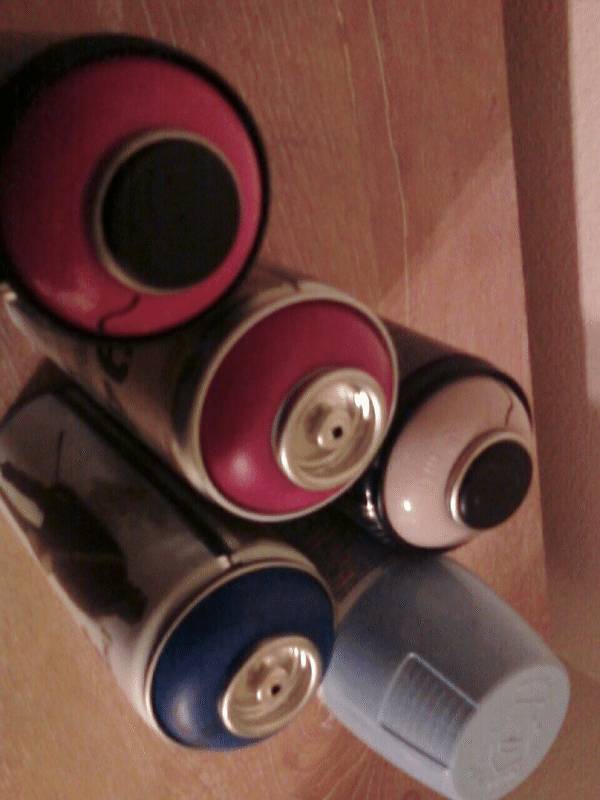This is an indoor, low-quality, color snapshot photograph with a red tint, slightly tilted to the right. The image captures five spray paint cans placed on a light brown wooden table. The photograph is taken from above, giving a top-down view, and appears to be out of focus. The cans are grouped in the center of the image and reflect some light. Out of the five cans, only one—located at the lower right—has a gray cap on, while the other four have their nozzles removed. The cans have a metallic exterior with their tops displaying concentric circles. The top left can features a hot pink or red top with a black circle in the center. The center can also has a hot pink or red top, but more of its silver body is visible. The can to the top right has a white top with a black circle. The bottom left can has a dark blue top with a silver circle, and the bottom right can, the only one with a cap, is light blue. The photograph is poorly lit, and no text or printing on the cans is legible. The angular orientation of the image makes the cans appear as though they are coming out of the wall.